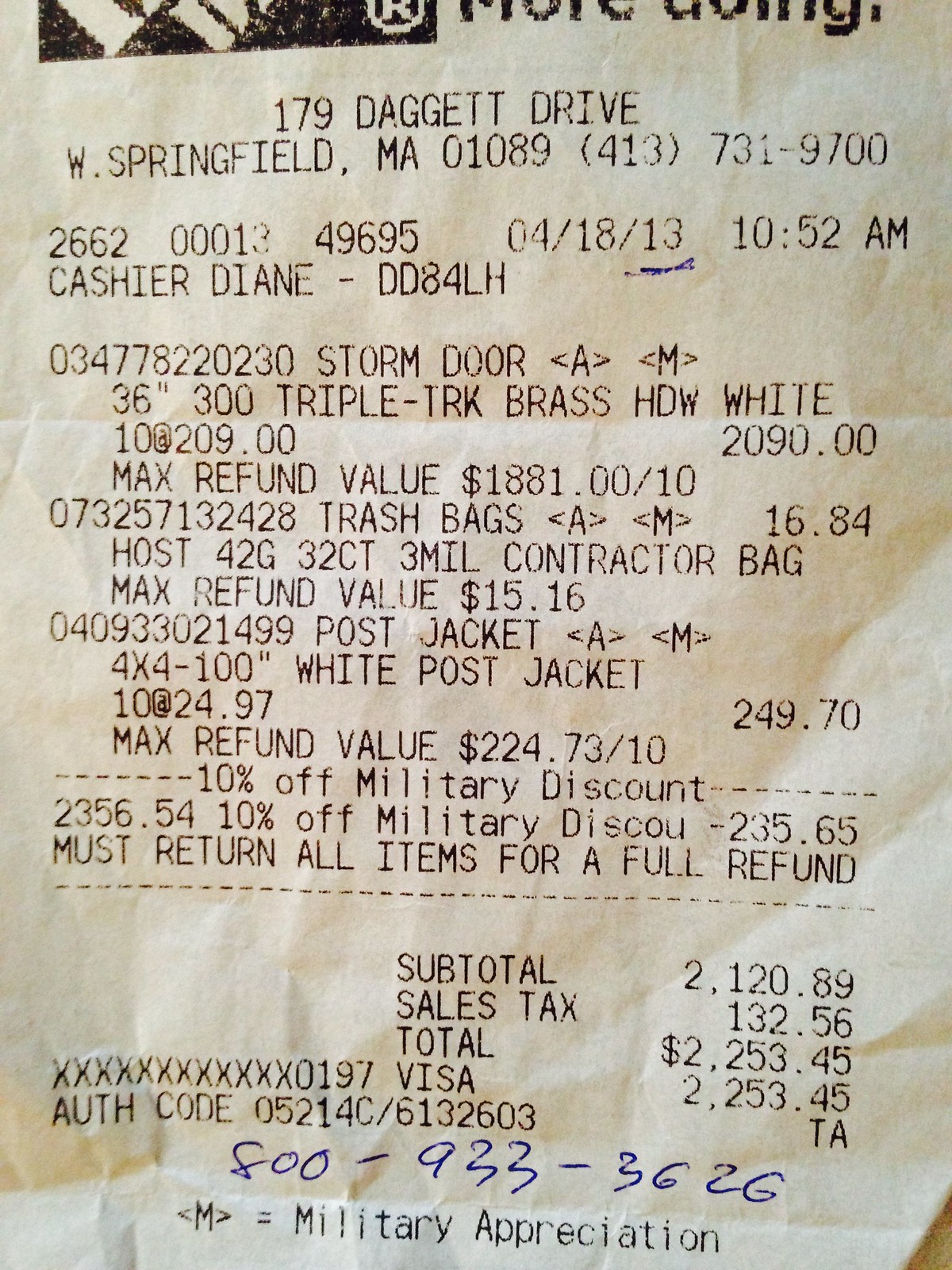The photograph captures a slightly crinkled, off-white receipt with black text, likely from a hardware store, possibly The Home Depot, as hinted by the partial logo and trademark on the upper right side of the receipt. The store's address "179 Daggett Drive, West Springfield, MA 01089" and phone number "413-731-9700" are prominently displayed. The purchase time is "10:52 AM" on "04/18/13," and the cashier identified is Diane, designated as "DD 84 LH." 

The itemized purchases include:
1. "Triple Brass HDW White" costing $2,090.
2. "Trash Bags" priced at $16.84.
3. "White Post Jacket, 4x4x100 inches" totaling $249.70.

Each item lists a refund value beneath it. The receipt mentions a "10% Military Discount" reducing the total by $235.65. The subtotal is noted as $2,120.89, with "Sales Tax" adding $132.56, bringing the full total to $2,253.45. Payment was made via Visa, confirmed by an authorization code "05214C/6132603." Additionally, there's handwritten blue ink at the bottom with the number "800-933-3626," followed by the notation "M = Military Appreciation."